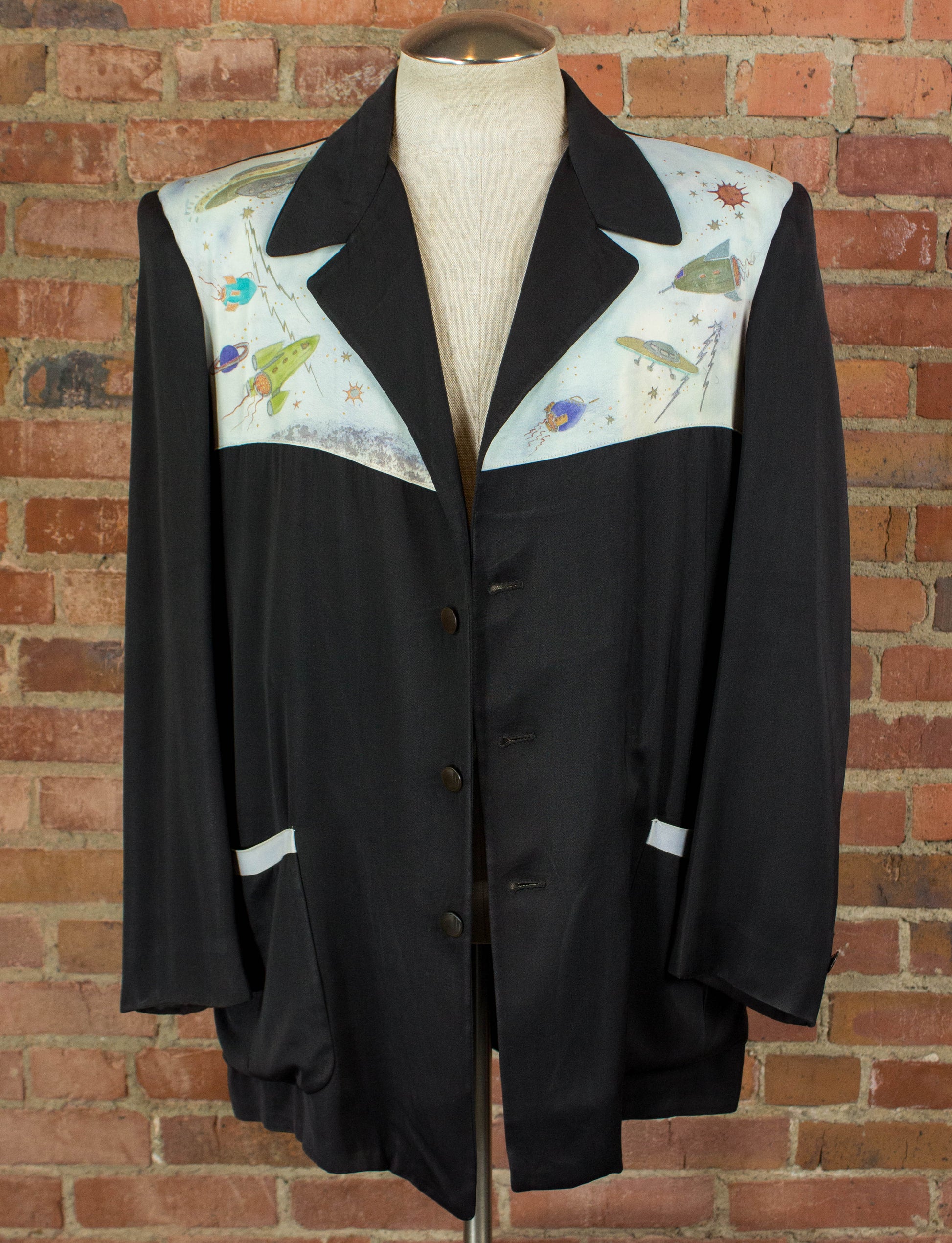Displayed against a red brick wall, this image captures a mannequin dressed in a unique black jacket. The mannequin is simple and designed to represent a male torso without a head or arms, supported by a long metal pole. The jacket is notable for its boxy fit and black notched lapels, featuring three large black buttons arrayed down the front. Long-sleeved with a button-up design, this garment has two pockets near the waist, each adorned with a white cuff at the top. The most striking feature of the jacket, however, is its whimsical yoke, which is light blue adorned with a playful alien-themed fabric. This fabric showcases a variety of colorful illustrations, including green and purple planets, blue and green rockets, flying saucers, and even a small depiction of Saturn with a yellow ring. The detailed imagery of spaceships, fire-emitting rockets, and extraterrestrial motifs adds a vibrant and imaginative touch to the otherwise sleek black jacket.